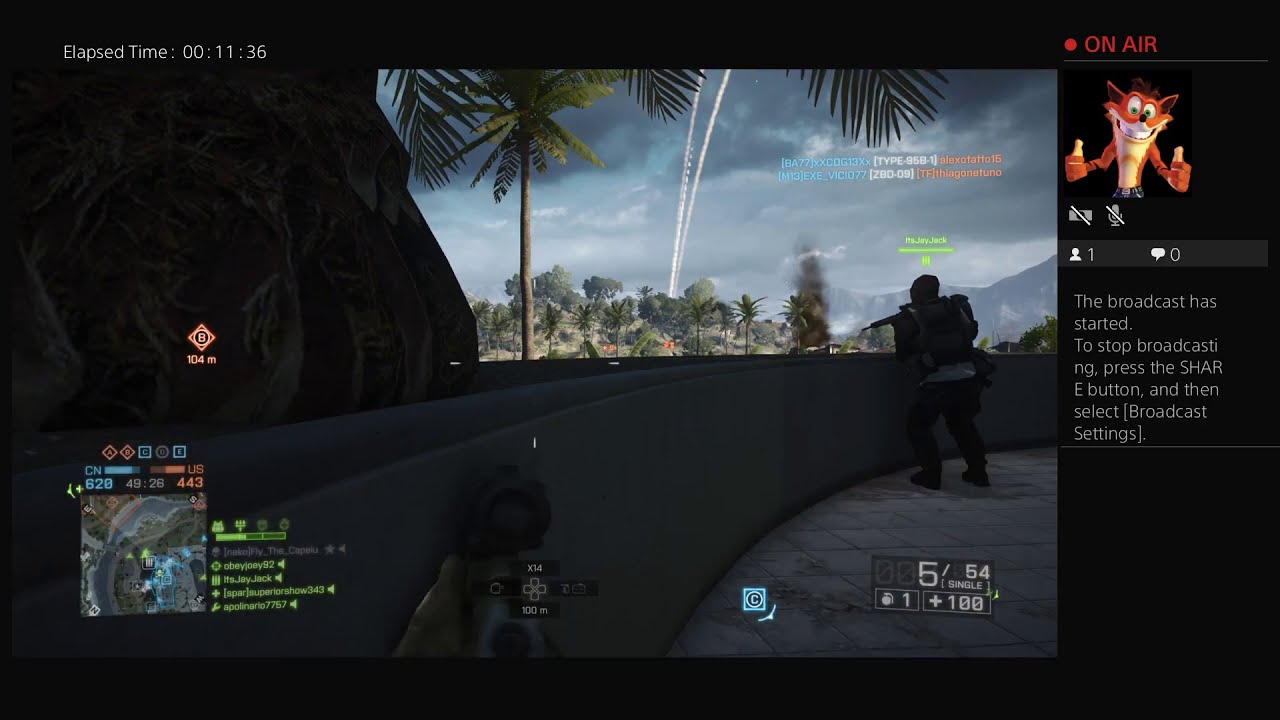The image captures a live broadcast of a first-person shooter game on PlayStation, potentially "Battlefield," with a predominantly black background. The top left corners display a white elapsed time of 11 minutes and 36 seconds, while the top right corner features a red "On Air" indicator. Just below this, there's an avatar of Crash Bandicoot giving two thumbs up, representing the gamer. Beneath the avatar, icons indicating that both the camera and microphone are off appear in gray. Further down, statistics show one viewer and zero comments, accompanied by white text stating, "The broadcast has started. To stop broadcasting, press the SHARE button and then select broadcast settings."

The left side of the image displays the game, set in a lush, tropical environment with green palm trees, likely resembling the Bahamas. Visible are two armed characters, one aiming a sniper rifle from behind a wall and another positioned nearby. The bottom left corner includes a map of the game area along with various in-game statistics like player lives. In the bottom right corner, additional stats such as ammo count and player health are shown. The vertical black bar on the right side indicates the PlayStation streaming interface.